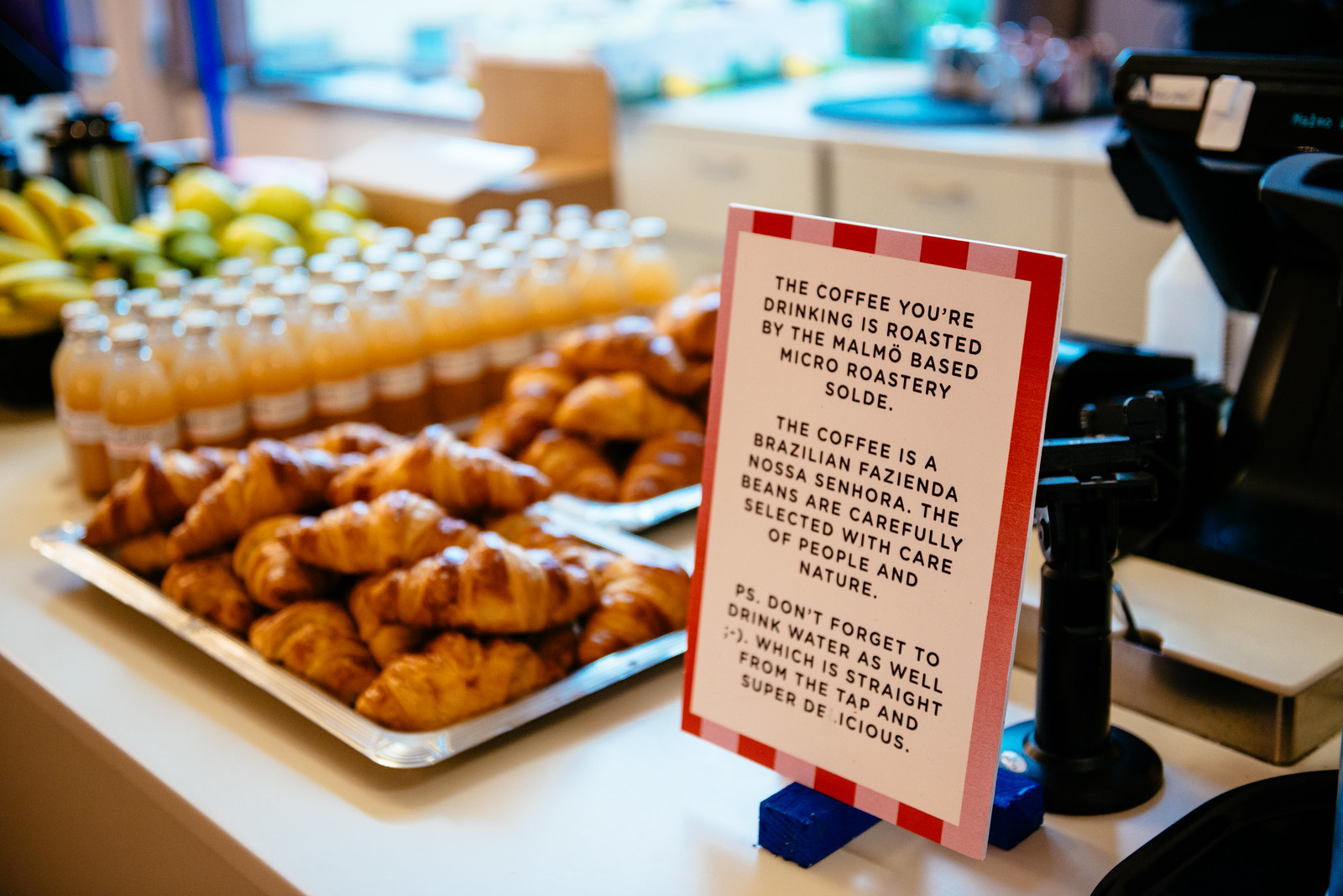The photograph is taken at a cozy bake shop counter featuring a variety of fresh items. On the right side, the back of a black cash register is visible. In front of the register stands a small sign on a blue stand, bordered with pink and red stripes against a white background. The black-font text on the sign reads: "The coffee you're drinking is roasted by the Malmo-based micro roastery Sold. The coffee is a Brazilian Fazenda Nossa Senhora. The beans are carefully selected with care for people and nature. P.S. Don't forget to drink water as well, which is straight from the tap and super delicious!" 

To the left of the sign, two trays overflowing with freshly baked, brownish-yellow croissants are prominently displayed. In front of these trays, there are several rows of bottles filled with what appears to be freshly pressed orange juice, their tops being either silver or white, and labels adorning the front. Further left, a bunch of yellow and green bananas peek from behind the juice bottles. In the background, there are tan and white walls along with white cabinets and drawers. A blue tray on the drawers holds indistinguishable items due to blurriness. Additionally, a brown cardboard box can be seen in the back. The overall setup is arranged on a white counter, giving the space a clean and inviting look. A silver coffee cup is also visible behind the bananas, adding to the culinary display.